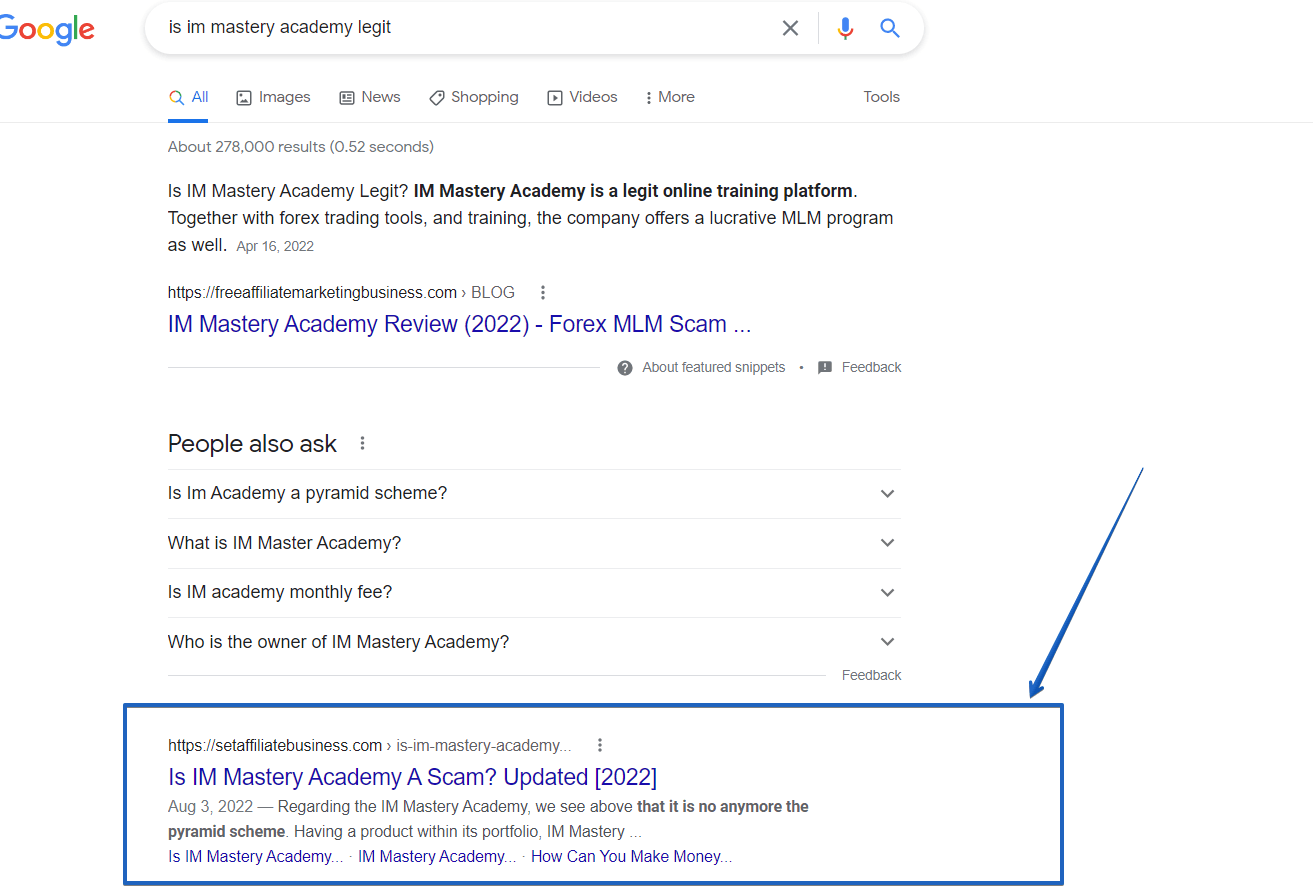An individual conducted a Google search to determine if IAM Mastery Academy is legitimate, using the query "Is IAM Mastery Academy legit?" One of the top search results featured the bold statement, "IAM Mastery Academy is a legitimate online trading platform." This result also highlighted the academy's offerings, which include Forex trading tools, training, and a multi-level marketing (MLM) program. Despite this affirmation, skepticism arises because MLM programs often have a reputation for being scams. The credibility of the information is further questioned by its source, "FreeAffiliateMarketingBusiness.com," which lacks reliability.

Additionally, Google’s "People also ask" section raises more inquiries about IAM Mastery Academy, including whether it's a pyramid scheme, the monthly fees involved, and details about the owner. Below this, another link titled "Is IAM Mastery Academy a scam? (Updated 2022)" appears, claiming that IAM Mastery Academy is no longer considered a pyramid scheme. However, given the source, this information remains dubious, reinforcing the impression that IAM Mastery Academy operates much like a pyramid scheme.